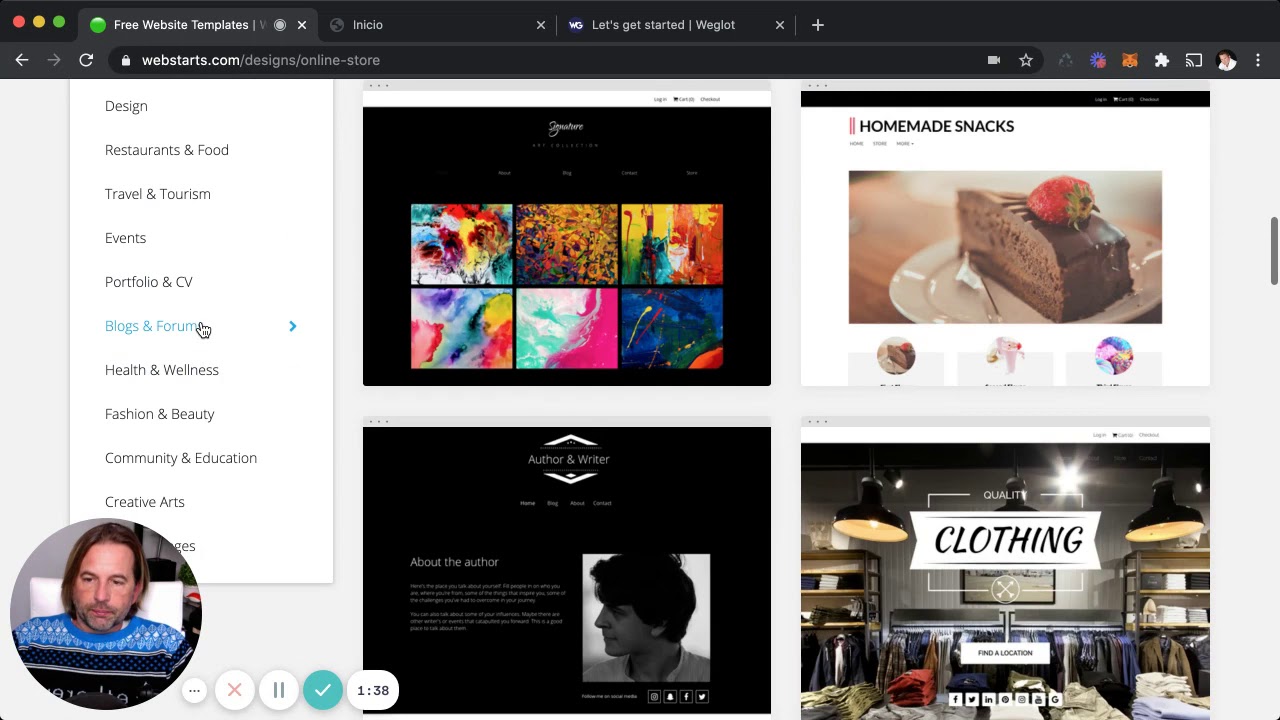A screenshot taken from a computer displays a search for "free website templates" in the search box. At the top, three browser tabs are visible: "INICIO," "Let's Get Started," and "WEGLOT." Below the search area, categorized sections for types of website templates are listed, including categories for "Design," "Restaurant and Food," "Travel and Tourism," "Events," "Portfolio and CV," "Blogs and Forum," "Health and Wellness," "Fashion and Beauty," "Community and Education," and "Creative Arts." 

In the upper right corner, a profile picture of a man is encircled; he has shoulder-length brown hair, a beard, and a mustache. He is wearing a blue and black sweater and has selected the "Blogs and Forum" category. To the right side of the screen, there is a square box featuring six thumbnails of abstract art. Adjacent to this box is an image captioned "Homemade Snacks," showcasing a delectable piece of chocolate cake on a white saucer, topped with a red strawberry.

In the bottom left corner beneath the thumbnails, another small thumbnail features a man's photo accompanied by the text "Author and Writer" and "About the Author," although the remaining print is too small to decipher. The final image to the right is labeled "Quality Clothing, Find a Location" and depicts numerous racks filled with men's shirts and shelves stacked with folded shirts.